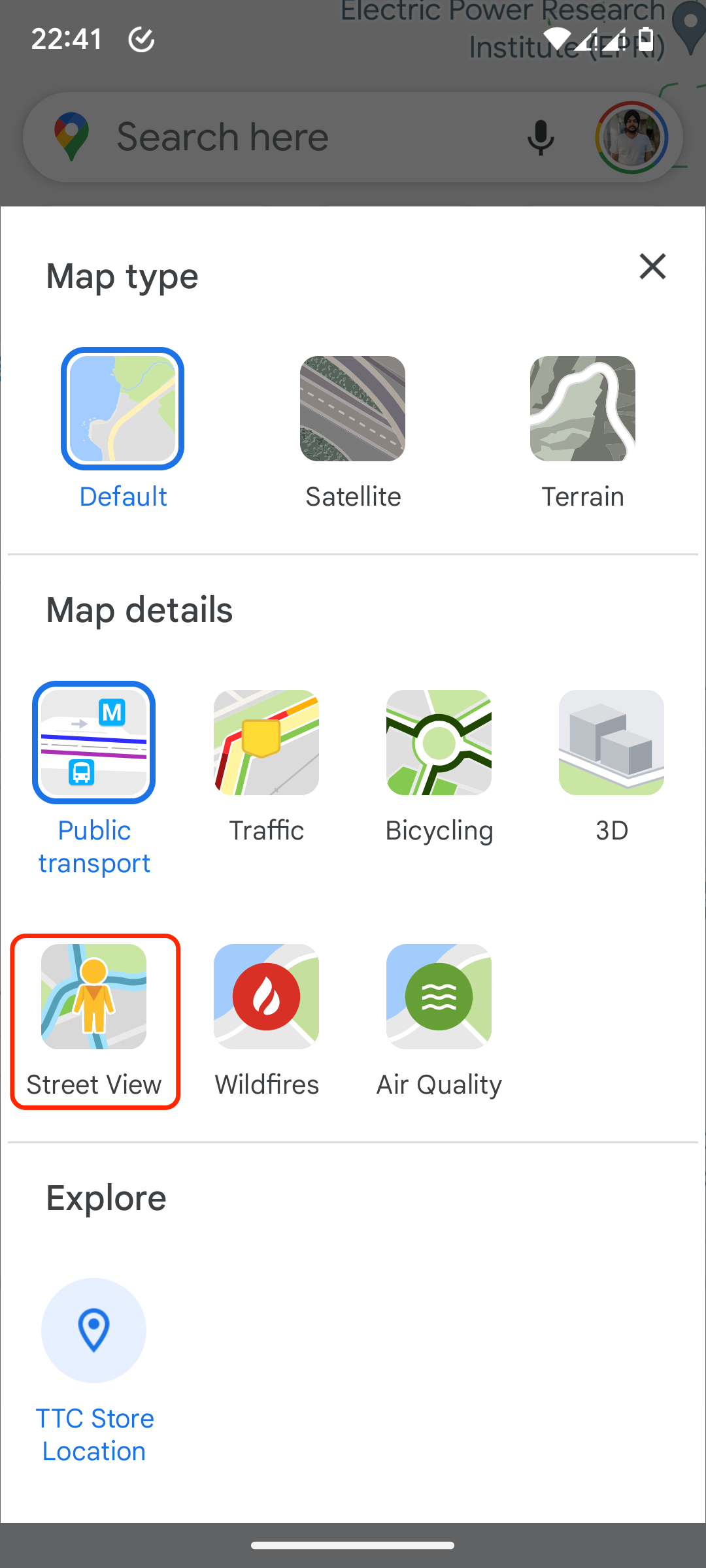This image is a detailed screenshot of a smartphone displaying an active Google Maps session, specifically showcasing a customization pop-up window. Through the transparent overlay, one can discern the Google Maps interface in the background, characterized by its dark gray theme. Prominently visible is the familiar Google Maps search bar, marked with a pin drop logo, microphone icon, and the user's Google profile picture on the right side. Behind the pop-up window, part of a pin drop indicating the "Electric Power Research Institute" is evident, affirming that the underlying layer is a functional map.

The customization pop-up itself is organized into three distinct sections: "Map Type," "Map Details," and "Explore." In the "Map Type" section, users have the option to select between "Default," "Satellite," or "Terrain" views, with each option accompanied by illustrative thumbnails. The "Default" option is currently selected, denoted by a blue border and blue font.

Moving to the "Map Details" section, there are multiple layers that users can toggle, including options for public transport, traffic, bicycling routes, 3D views, street view, wildfires, and air quality indicators. Presently, the "Public Transport" layer is activated, as highlighted by a blue banner. A red square over the "Street View" button suggests it is being considered for activation next.

The final section, "Explore," features a single pin drop icon paired with the label "TTC SOAR location," indicating a specific point of interest. This comprehensive screenshot encapsulates the extensive customization capabilities within the Google Maps application, offering a detailed glance at the various layers and viewing options available to users.